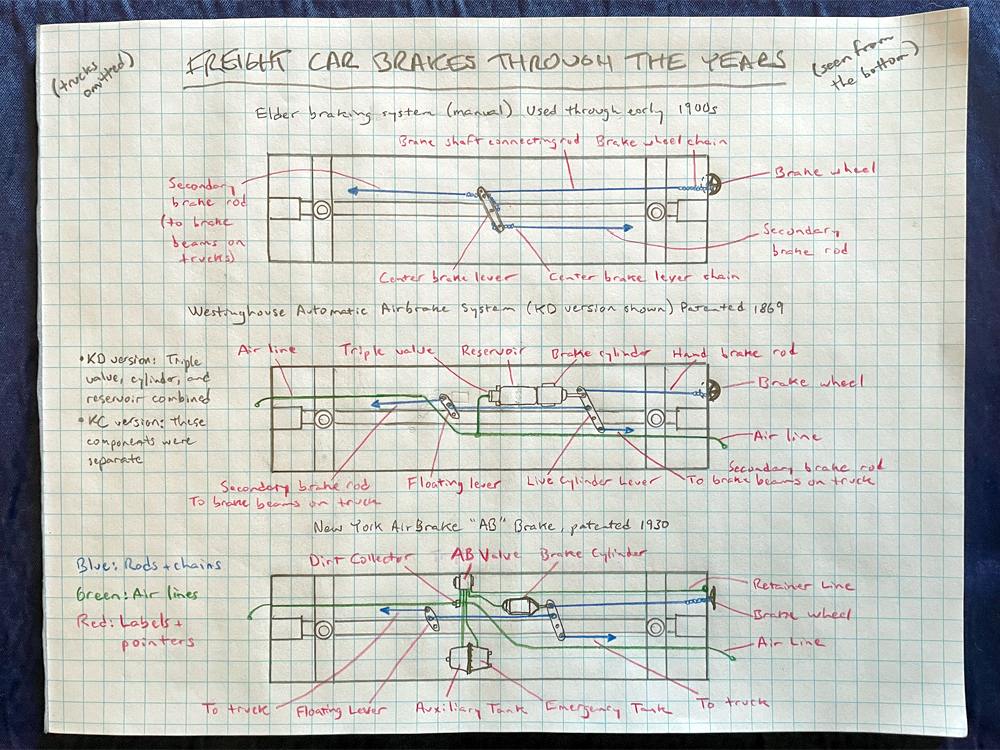This photograph vividly captures a detailed and densely annotated schematic drawn on a piece of graph paper, characterized by small, thin blue lines forming a meticulous grid. The paper rests on a dark blue fabric surface which darkens toward the bottom part of the image. At the very top of the graph paper, in neat, capital gray pencil lettering, it reads "FREIGHT CAR BREAKS THROUGH THE YEARS," flanked on the left by the note "(trucks omitted)" and on the right by "(seen from the bottom)." 

Beneath this title, three wide rectangular graphs are methodically illustrated. The first graph is labeled "Elder Braking System (Manual, Used Through Early 1900s)," written in subdued gray. The second graph is titled "Westinghouse Automatic Air Brake System (KD version shown, patented 1869)," while the third graph is identified as "New York Air Brake, AB Brake (Patented 1930)." Each graph reveals a complex system where various lines (green and blue) and red ink indicate different components, all meticulously labeled with red pens and arrows pointing to each part. 

Additional notes are interspersed throughout the document, marked by asterisks on the left side. In the bottom left corner, a key decodes the colors: "Blue, Red, and Chains; Green, Airlines; Red, Label and Pointers." This key clarifies the purpose of the different hues. Despite the myriads of labels and pointers, the intricate care in the drawing and annotation stands out, making it a well-crafted illustration rich in historical railway braking system details.